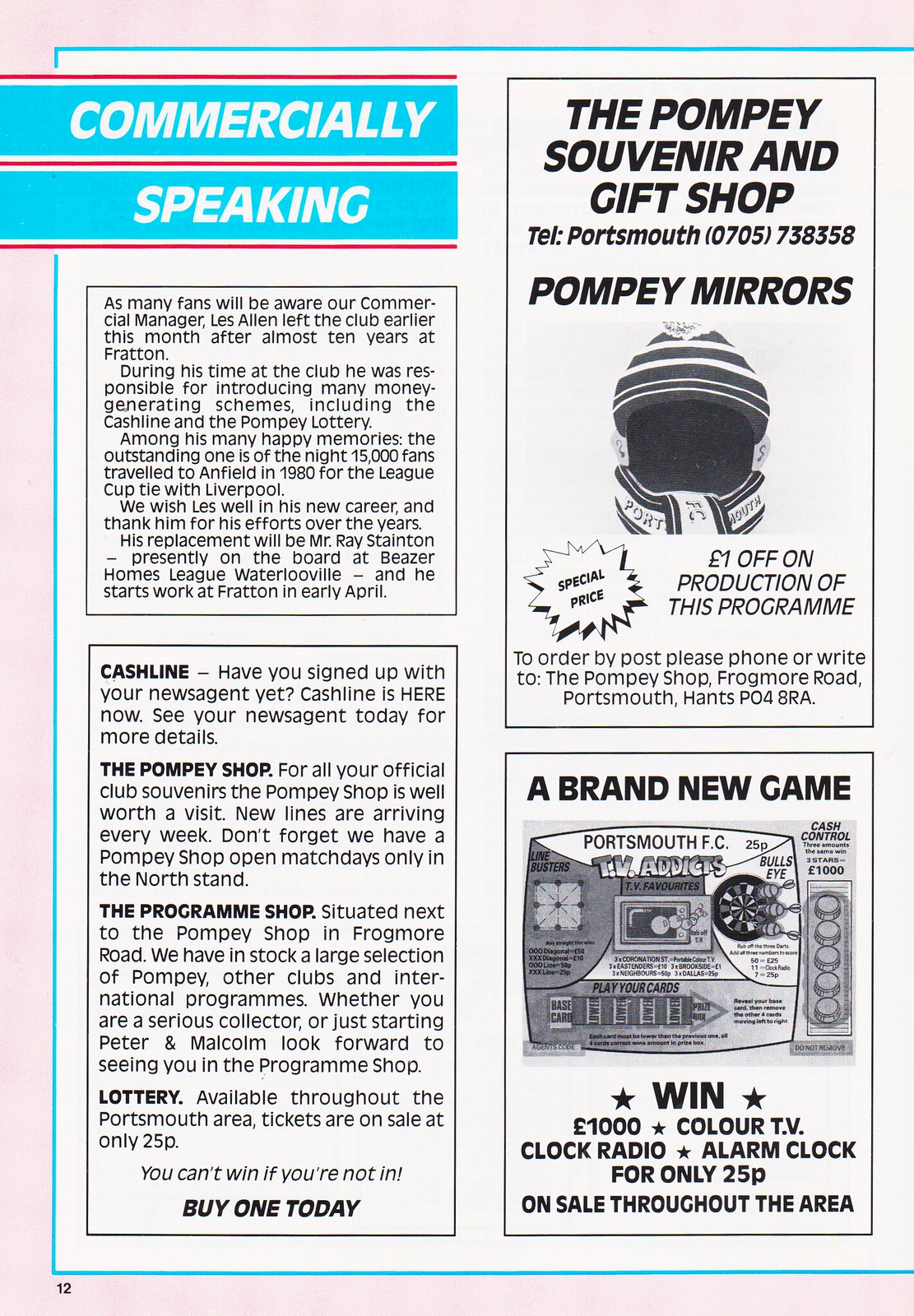This image is a dated screenshot, possibly from the 80s or 90s, showing page 12 of a magazine or newspaper. The title "Commercially Speaking" is prominently displayed in light blue and white letters with three separating red lines across the page. The layout includes multiple advertisements in black and white, interspersed with sections of light blue and pink shading.

The top right corner features an advertisement for the Pompey Souvenir and Gift Shop, which highlights Pompey Mirrors and includes a telephone number for orders. There's an intriguing image of a person with their face blacked out, wearing a beanie and scarf. Below this, it offers a £1 discount on the production of this program, accompanied by a mailing address for the shop in Portsmouth.

The bottom right corner of the page advertises a brand new game with a raffle that boasts prizes including £1,000, a color TV, a clock radio, and an alarm clock, all available for just 25 pence. This ad beckons readers to win big with its bold "WIN" announcement and star accents.

On the left side of the page, more commercial descriptions are detailed in text, including mentions of Cashline, the Pompey Shop, the Program Shop, and a Lottery, encapsulated with the tagline "Buy One Today." There are also light blue rectangles labeled "commercially" and "speaking."

Overall, the page captures a nostalgic glimpse into past advertising styles, complete with specific offers and promotional content aimed at drawing in readers for various local shops and contests.